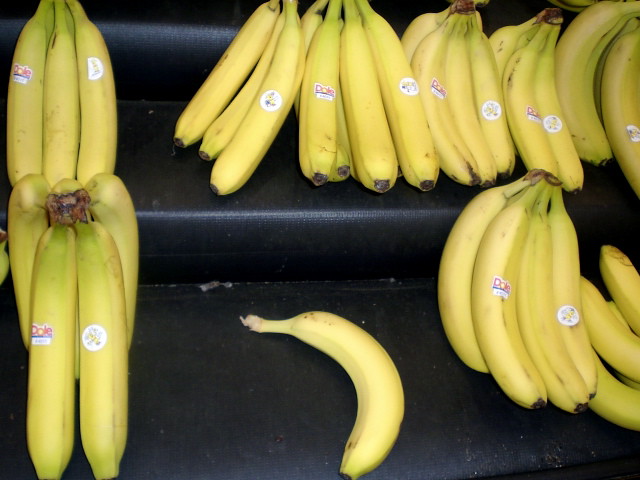A vibrant display of Dole brand yellow bananas is neatly arranged on a layered black shelving unit within a grocery store. The tiered structure consists of three steps, each ascending higher from bottom to top, ensuring all bananas are easily visible to shoppers. While the shelving is only partially filled, it effectively showcases the ripe, yellow fruits.

On the topmost visible shelf, only a fragment is shown, leaving the exact banana count uncertain. The second shelf down, nearly full, holds six bunches of bananas, each varying from three to six per bunch. These bananas exhibit a vibrant yellow hue with faint green at the stems and brown tips at both ends, indicating their ripeness. Not every banana has a sticker, but each bunch features two prominent labels: one side boasts the recognizable Dole logo in red and blue, while the other displays a circular white sticker adorned with an indistinct image. A noticeable gap appears near the left side of this otherwise densely packed shelf.

The bottommost visible shelf is sparsely populated. To the far left, a clump of five bananas stands alone. Adjacent to this grouping is a stretch of empty black shelf, interrupted by a solitary banana lying on its side, gently curving left. Towards the right end, two additional clumps of bananas complete the display. The arrangement, though not entirely filled, highlights the freshness and appealing presentation of the bananas for potential buyers.